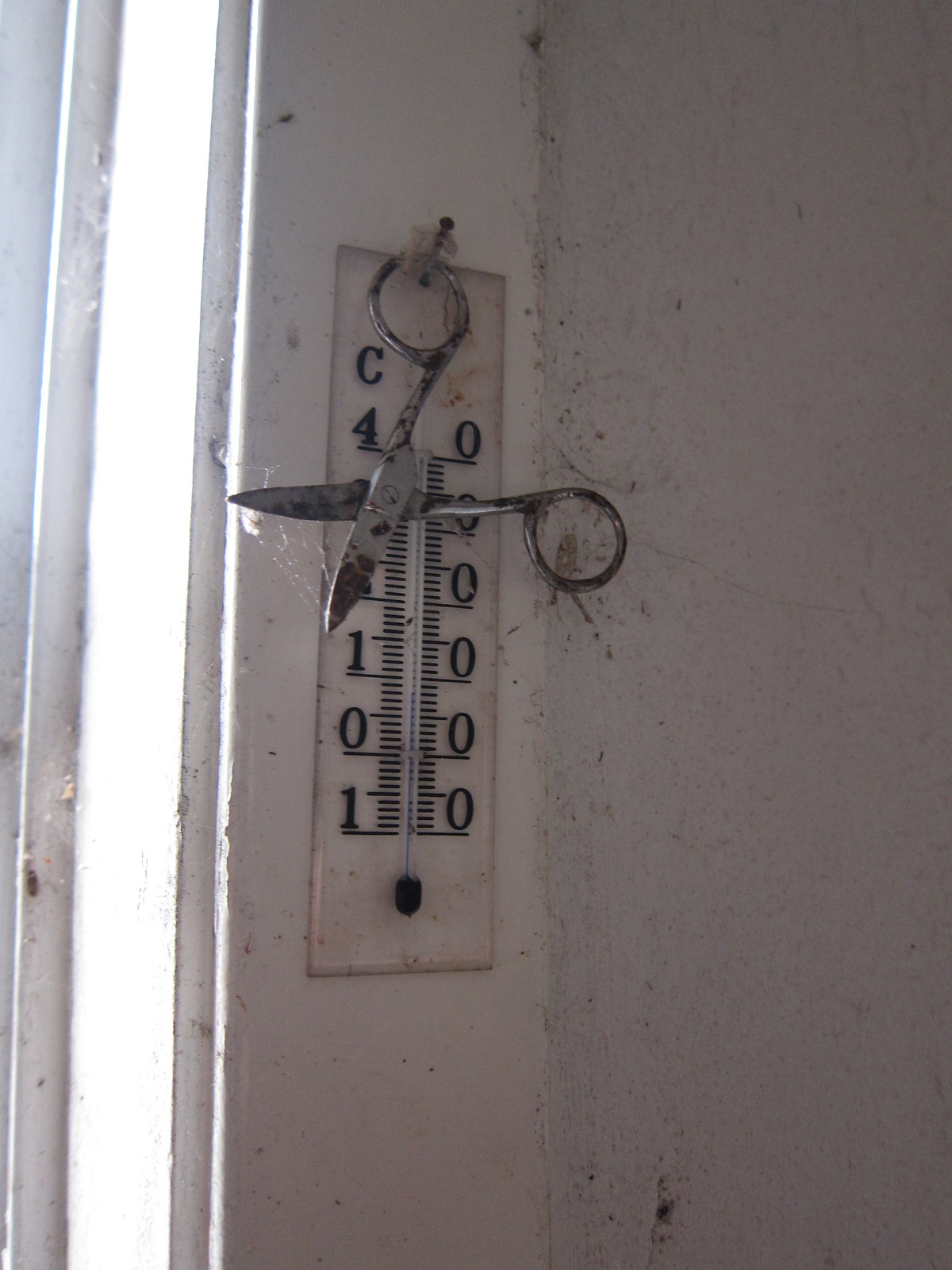This photograph presents an intriguing scene featuring a white wall corner of a building, which shows signs of aging and wear, marked by black and brown stains. Attached to this wall is a nail that holds both a thermometer and a pair of old, rusted metal scissors. The thermometer, about one to two feet in length, appears to use mercury to display temperatures. Its scale is somewhat discernible with numbers likely indicating 40, 30, 20, 10, 0, and -10 degrees, marked in descending order and interspersed with smaller markers indicating increments of 5 degrees. The door frame in the background, possibly belonging to a screen door, is open, further adding to the aged and potentially abandoned ambiance of the setting.